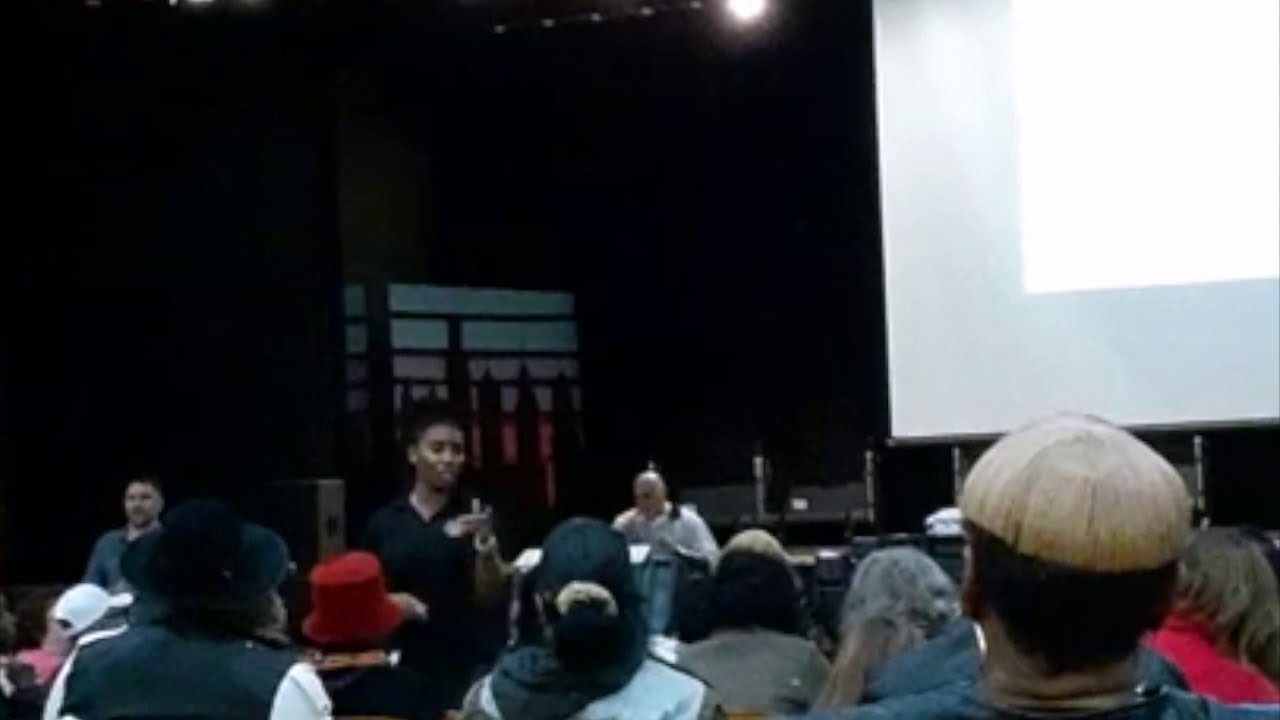The slightly blurry, low-resolution photograph captures the back view of an attentive crowd, mostly sitting, with a variety of hair colors and some wearing hats. They focus on a young African American woman with dark hair in a black shirt who stands slightly left of center, her arm raised as if presenting something to the audience. Toward the center of the image, a man in a white shirt, possibly a security guard, stands, while another person dressed in black is positioned further to the left. The backdrop is predominantly dark, suggesting an indoor setting, illuminated by lighting from above. To the left of center, a vibrant piece of artwork or window features blue, purple, and pink stripes. The top right corner of the image reveals a large white area likely serving as a projector screen, contributing to the suggestion of a staged event like a meeting, rally, or presentation. The scene is punctuated by the varied attire of the crowd, including jackets and casual wear, with the occasion possibly being an activist meeting or a Q&A session.